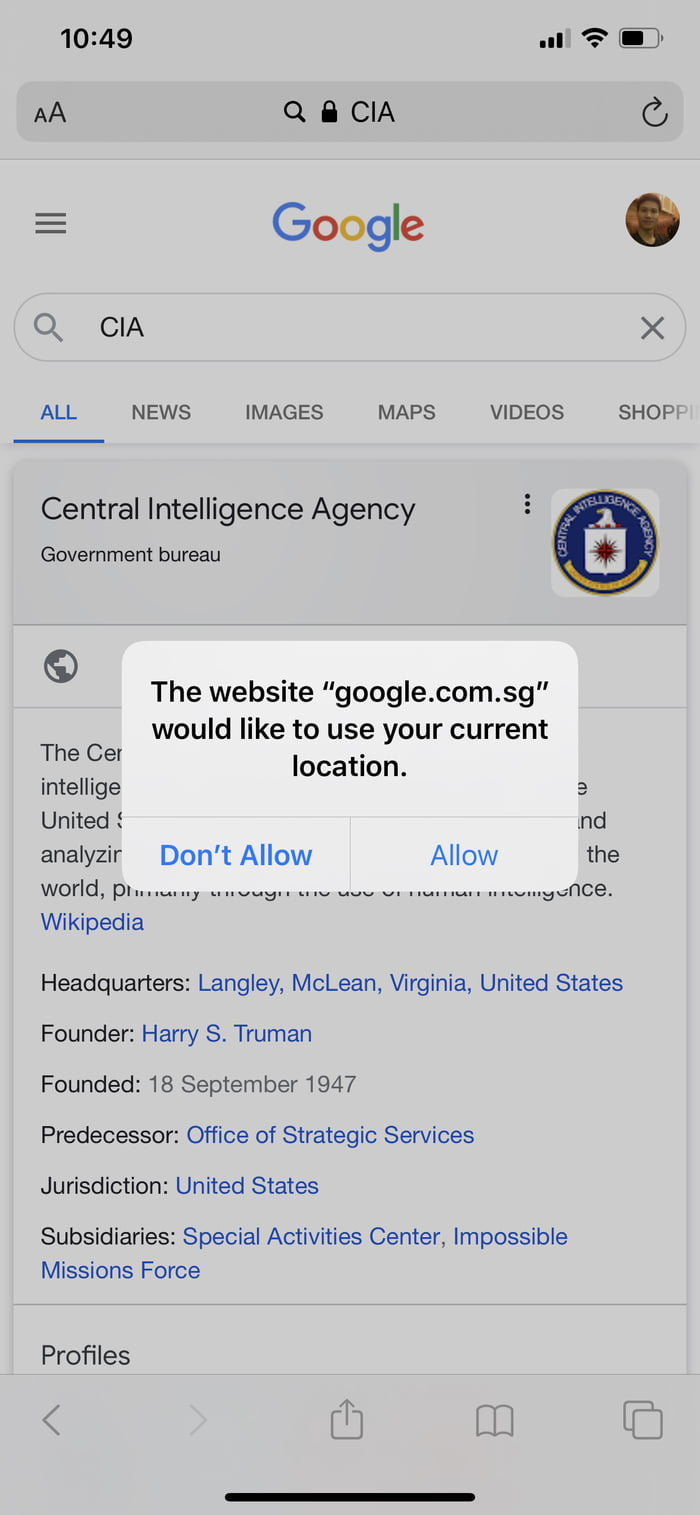A smartphone screen is displayed with a pop-up notification overlaying the main webpage. The pop-up, a small green rectangle with black text, states: "google.com.sg would like to use your current location." Below the message is a horizontal gray line, beneath which are two options: "Don't Allow" on the left, highlighted in blue, and "Allow" on the right.

In the backdrop, the main page has dimmed, but some details are still visible. At the top of the screen, indicated in black, it's 10:49 AM, and the device shows a strong Wi-Fi connection with four bars and decent cell reception with three out of four bars.

The webpage appears to be a search result for "CIA" on Google. At the top of the webpage, there is a gray rectangular bar with "CIA" written in black. To the left of this text are three horizontal gray lines, likely indicating a menu. Centered at the top is the Google logo in its signature colors: red, blue, yellow, blue, green, and red. Adjacent to the logo, there’s a profile picture, though the details are indeterminate. Below the search bar, outlined in gray and featuring a magnifying glass icon and the text "CIA," there's a small 'X' button for clearing the search.

Beneath the search bar, a navigation bar displays multiple tabs. Most tabs, such as "News," "Images," "Maps," "Videos," appear in gray, but the "All" tab is blue, indicating it's the active selection. The visible search result is a detailed entry for the Central Intelligence Agency (CIA), providing information about its headquarters in Langley, McLean, Virginia, USA, its founder Harry S. Truman, its founding date of September 18, 1947, its predecessor the Office of Strategic Services, its jurisdiction, and subsidiaries including the Special Activities Center and the Impossible Missions Force.